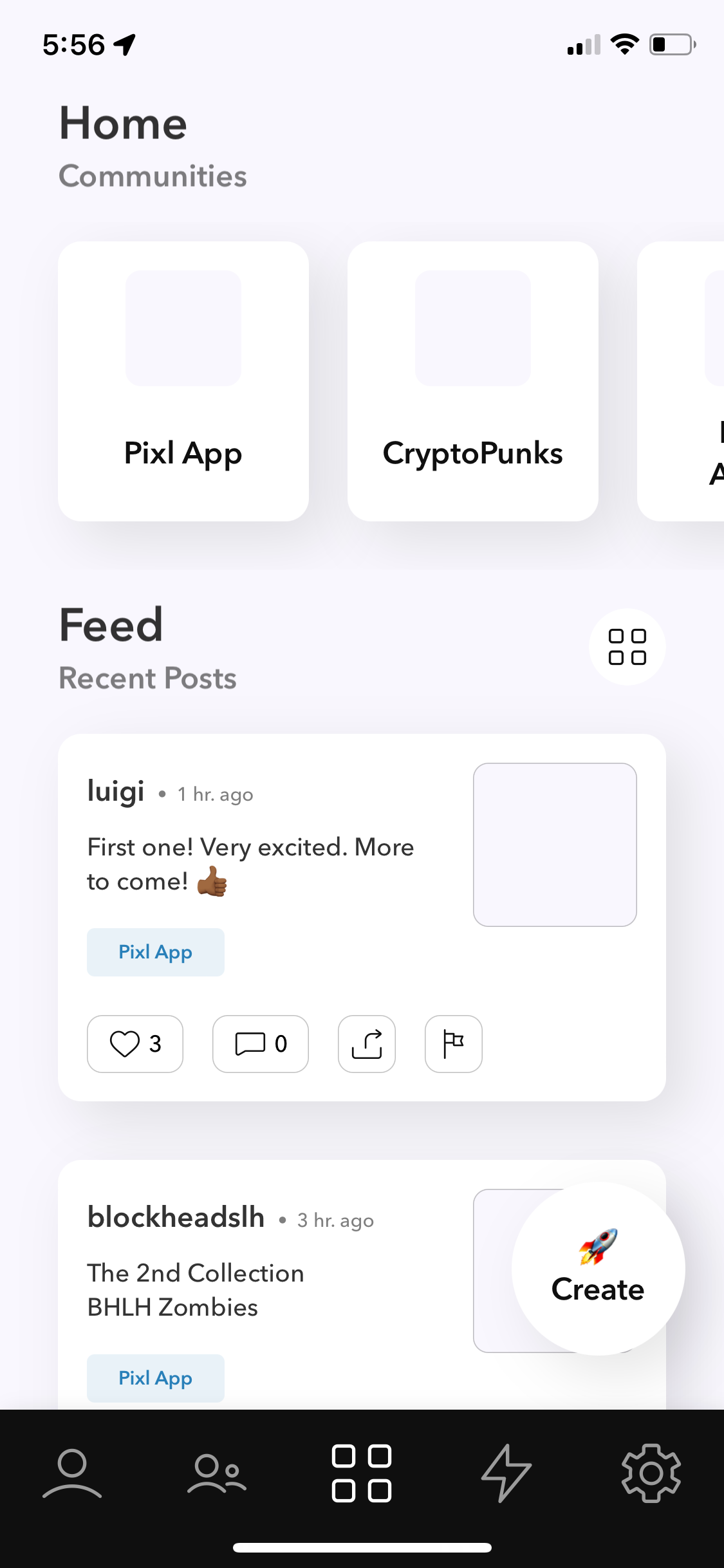This image is a mobile screenshot of the GrinGo app, featuring a white background. In the bottom-right corner, there's a round button with a rocket icon labeled "Create," indicating it’s GrinGo's distinctive feature. 

At the top-left corner of the screen, the word "Home" is prominently displayed in black letters. Beneath "Home," the word "Communities" appears in gray. 

The app also features two interactive boxes at the top, labeled "Pixel App" and "CryptoPunks," though their thumbnails are missing. These boxes can be scrolled horizontally, and part of another box is visible on the right edge.

Below the community boxes, the section is titled "Feed" in bold black letters. Underneath that, "Recent Posts" is mentioned in small gray letters. Here, the app displays posts within white boxes.

The first post shown is by a user named Luigi, marked as posted one hour ago. Luigi’s post reads, "First one, very excited, more to come." Below this text, there’s a button labeled "Pixel App," with a missing thumbnail to the right. At the bottom of Luigi’s post, there are options to like, comment, share, or flag the content.

The second visible post, located beneath Luigi’s, is by a user named BlockheadsLH, posted three hours ago. The post states, "Second collection, BHLHzombies," followed by a button labeled "Pixel App."

This detailed layout gives a comprehensive view of the GrinGo app's interface and features.